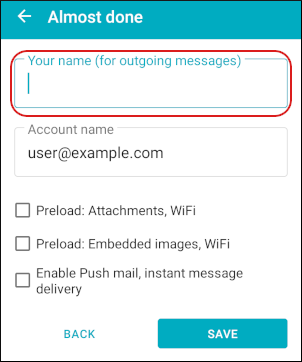This is a screenshot of a pop-up menu from a website or app, featuring various settings and input fields. At the top, there is a light greenish-blue bar with a white left-pointing arrow icon next to the text "Almost done," also in white font. Below this bar is a white rectangular area. 

The first section within this area is a gray rectangle labeled "Your name (for outgoing messages)." Below this label is an empty text field indicated by a blinking cursor, and this field is circled in red for emphasis. 

The next section is another text field labeled "Account name" in gray, with the placeholder text "user@example.com" displayed inside it.

Further down, there are three checkbox options for different settings:
1. "Preload: attachments, WiFi"
2. "Preload: embedded images, WiFi"
3. "Enable pushmail, instant message delivery"

At the bottom of the white rectangle, on the right side, there is a blue button labeled "Save" in white text. On the left side, there is a blue text link labeled "Back."